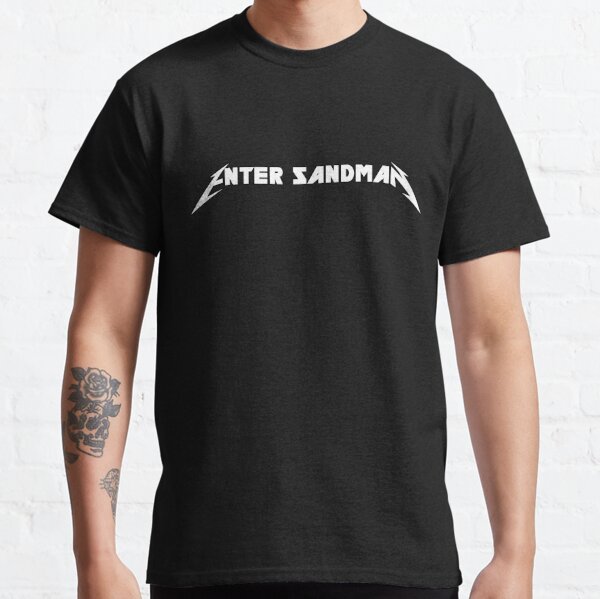In this detailed image, a young, presumably white, man is photographed against a white brick wall background, which has been painted over. He is wearing a black t-shirt emblazoned with the words "Enter Sandman" in white letters, a nod to Metallica's iconic song. The "E" of "Enter" and the "N" of "Sandman" are stylized differently, reminiscent of the Metallica band logo. The shirt is otherwise simple, with no additional designs. The man's right arm is adorned with tattoos, including a skull and a rose; there also appears to be another, less discernible tattoo near his wrist. The left arm has no visible markings. The photo's framing excludes his face and any part of his body below the t-shirt.